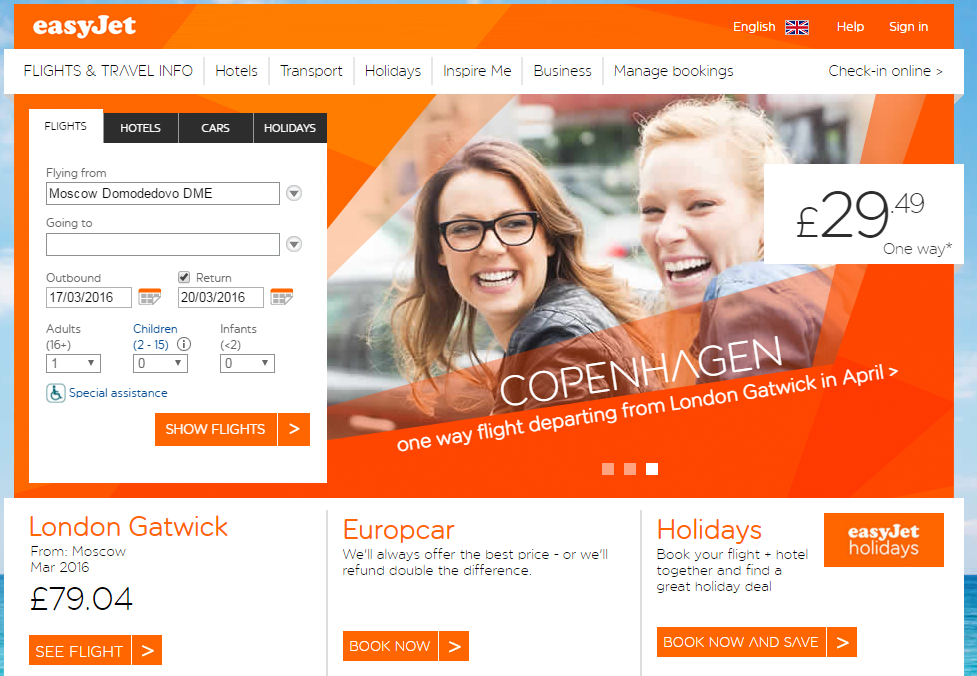### Detailed Caption for EasyJet Website Screenshot

This image captures a screenshot of EasyJet's website. The webpage design features a light blue background at the edges, evoking a bright sunny sky with scattered clouds and a hint of ocean at the bottom corners. Dominating the page is an orange box with gradients that transition from darker orange to lighter shades and back.

**Header Details:**
- **Top Left:** The EasyJet logo in bold white letters, with "easy" in lowercase and "JET" in uppercase.
- **Top Right:** 
  - "English" followed by a UK flag.
  - "HELP" in white.
  - "SIGN-IN" in white.

A white banner below the header offers a series of menu options:
- **Flight & Travel Info** in uppercase.
- **Hotels, Transport, Holidays, Inspire Me, Business, Manage bookings**
  - Note: "Manage bookings" has only "Manage" capitalized.
- **Check-In Online** accompanied by a right-pointing triangle symbol.

**Main Search Section:**
On the left side, there’s a tabbed search box:
- **Tabs:**
  - "FLIGHTS" highlighted in white.
  - "HOTELS," "CARS," and "HOLIDAYS" in black text on white.
- **Flight Search Fields:**
  - **Flying From:** Pre-filled with "Moscow, Domodedovo (DME)" and a dropdown icon.
  - **Going To:** Empty text box with a dropdown icon.
  - **Dates:**
    - **Outbound:** Filled with "17-03-2016" alongside a calendar icon.
    - **Return:** Checked with a date "20-03-2016," a calendar icon, and an optional checkbox.
  - **Passenger Information:**
    - **Adults (16+):** Dropdown box with "1" selected.
    - **Children (2-15):** Dropdown box set to "0," with an info icon.
    - **Infants (<2):** Dropdown box set to "0."
  - **Special Assistance:** Indicated by a green handicap icon and a blue "SPECIAL ASSISTANCE" label.
  - **Search Button:** A bright orange "SHOW FLIGHTS" button with a right-pointing symbol.

On the right side, a picture of two smiling, glasses-wearing Caucasian women is shown. Below it:
- **Destination:** "COPENHAGEN" in white text on an orange translucent banner.
- **Price Badge:** White badge with "GVP 29.49."
- **Flight Details:**
  - "ONE WAY" with an asterisk.
  - "COPENHAGEN," followed by "ONE WAY FLIGHT DEPARTING FROM LONDON GATWICK IN APRIL" and an arrow.
  - Navigation dots below the text, indicating the first dot is selected.

**Bottom Sections:**
1. **Left Section:**
   - Orange label: "London Gatwick"
   - Black text: "from Moscow,"
   - Date: "Mar 2016"
   - Price: "GVP 79.04"
   - Orange button: "SEE FLIGHT" with a right-pointing arrow.

2. **Middle Section:**
   - "EUROPCAR" in orange.
   - Black text: "WILL ALWAYS OFFER THE BEST PRICE - OR WILL REFUND DOUBLE THE DIFFERENCE."
   - Orange "BOOK NOW" button with a right-pointing arrow.

3. **Right Section:**
   - Orange label: "HOLIDAYS"
   - Black text:
     - "BOOK YOUR FLIGHT PLUS HOTEL TOGETHER AND FIND A GREAT HOLIDAY DEAL."
   - Orange badge: "EASYJET HOLIDAYS" in white.
   - White text on an orange button: "BOOK NOW AND SAVE" with a right-pointing triangle.

This comprehensive and structured description provides a detailed overview of the visual elements and content layout on the EasyJet website screenshot.